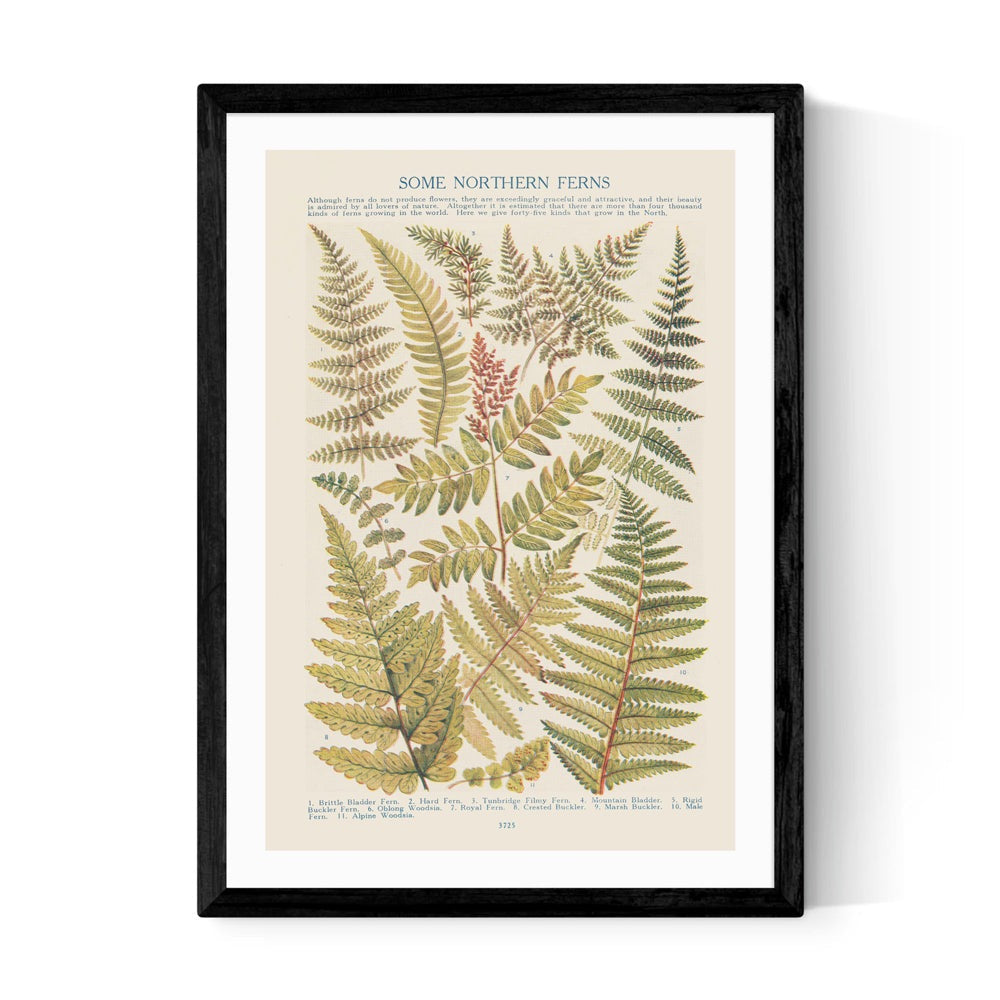This image features a black photo frame with an ivory background, inside which is a picture. At the top of the picture, there is text in blue that reads "Some Northern Ferns," followed by a few sentences describing them. The main section of the image showcases various types and sizes of green ferns, possibly numbering around ten, all depicted in similar shades of green. The background of the depicted photo is light brown with an additional white border around the edges.